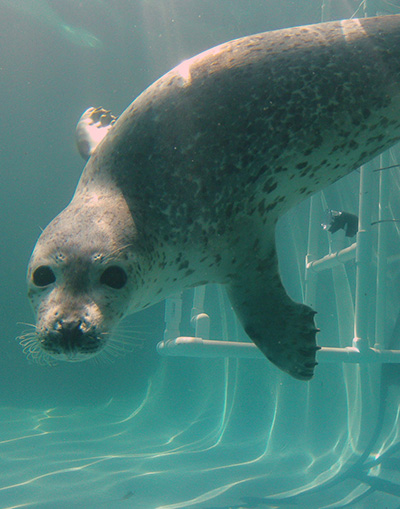The underwater photograph captures a grey, spotted seal swimming and looking straight at the camera with its large black eyes and whiskers clearly visible. The seal's body, dark on top and lighter underneath, is inverted as it dives, with its front limbs extended and its black nose pointing downward. Sunlight filters through the blue water, highlighting the artificial setting—possibly a pool or zoo enclosure—with visible white structures and rods in the background. The tank's bottom features what looks like pipes, emphasizing the man-made environment. Rays of sunlight illuminate the scene, emphasizing the seal’s graceful motion and natural curiosity as it seemingly swims towards the camera.